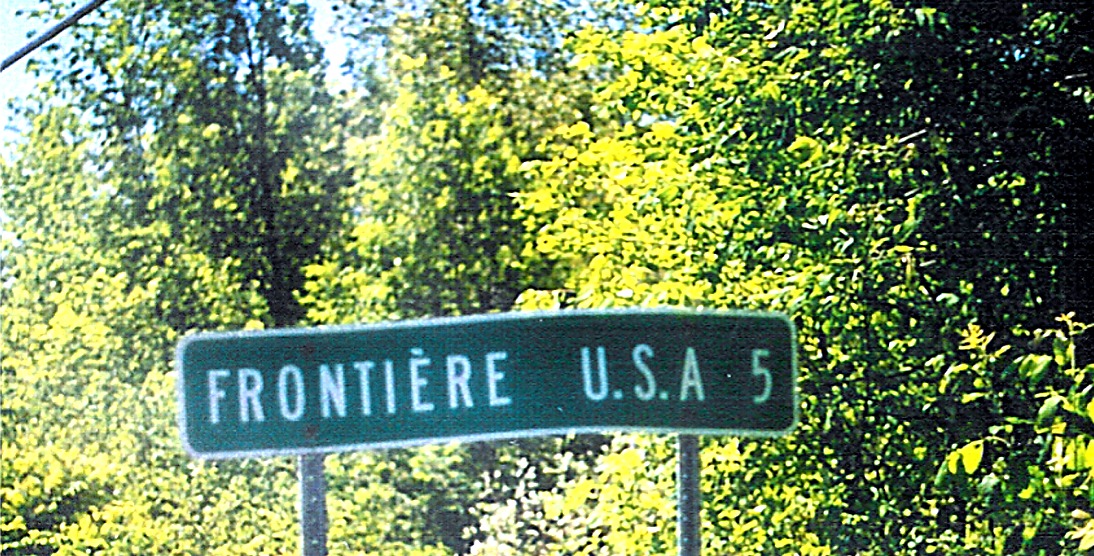The image depicts a road sign, predominantly dark green with white text and a white border. The sign reads "FRONTIÈRE U.S.A. 5" in all capital letters, with accent marks over the 'R' and 'E' in "FRONTIÈRE." It is supported by two slender, metallic poles on either side, giving the impression that it's securely grounded. The background showcases vibrant foliage, with varying shades of green from light to dark, capturing sunlight filtering through the trees. The sky in the top left is a light blue, marked by streaks of clouds. The right side of the image contrasts with more shadow, where the sunlight doesn't penetrate the dense tree cover as effectively. The image has a somewhat blurry and low-quality appearance, possibly indicating it was taken from inside a moving vehicle.